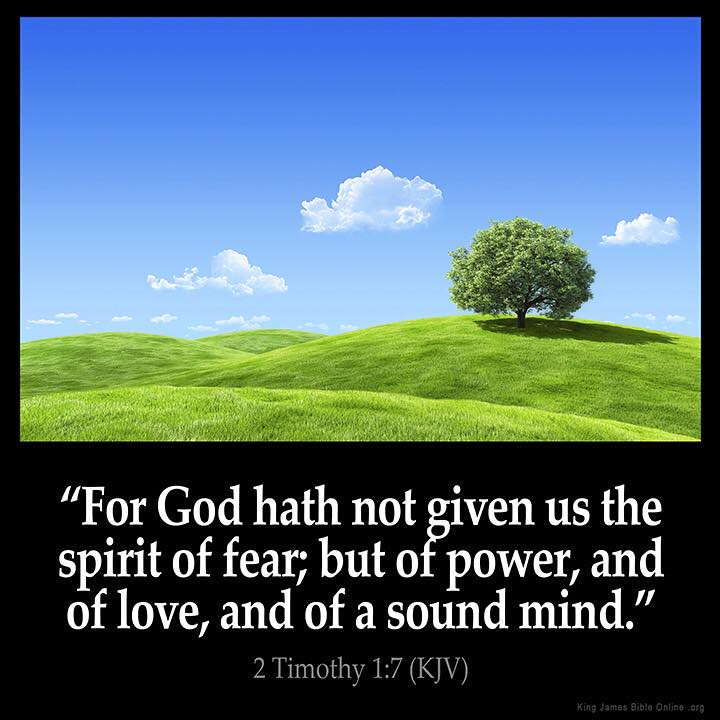The image portrays a serene landscape featuring rolling green hills covered in bright grass. On the right side, atop one of these hills, stands a solitary tree adorned with vibrant green leaves, casting its shadow on the ground. The sky above is a gradient of light to dark blue, populated with scattered white clouds. The composition occupies approximately the top two-thirds of the image, creating a tranquil and picturesque scene. Below this tranquil landscape, there's a black segment containing a Bible quote in bold white text: "For God hath not given us the spirit of fear, but of power, and of love, and of a sound mind. 2 Timothy 1:7 KJV." Additionally, the bottom right corner features the phrase "KingJamesBibleOnline.org," attributed to the source of the quote. This richly detailed image, likely created digitally, evokes a sense of calm and spiritual reflection.